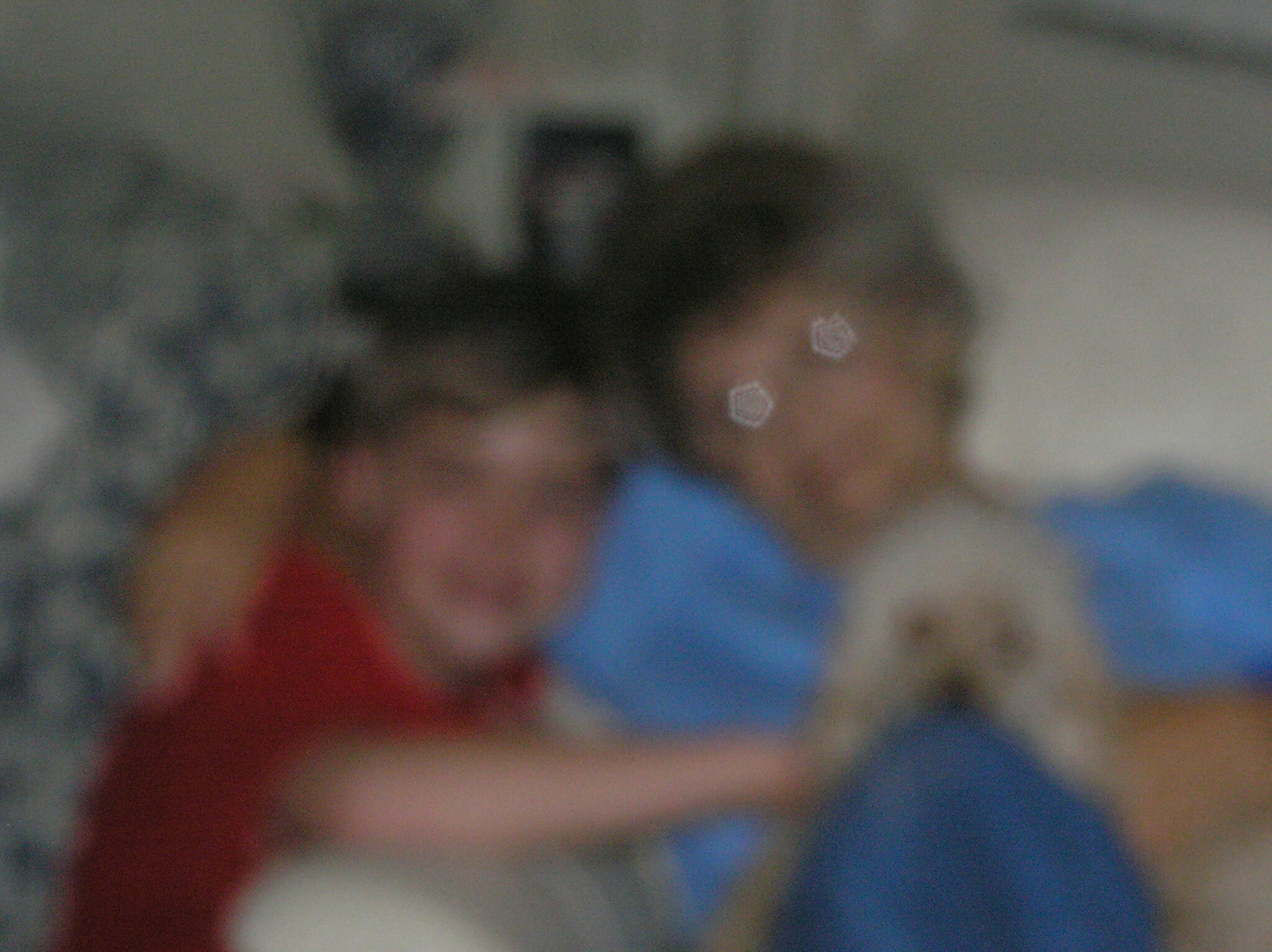In this image, an out-of-focus shot captures a heartfelt moment featuring a boy, a woman, and a dog. Despite the blur, the warmth of the scene is palpable. The dog, with its brown fur, gazes directly at the camera, exuding an innocent curiosity. Beside the dog, a woman, dressed in a blue shirt, appears to be refracting light, suggesting she’s wearing glasses. Her short brown hair frames her face. The boy, wearing a red shirt and seemingly smiling brightly, is gently petting the dog, adding a sense of affection to the composition. While the background is predominantly white, possibly indicating a wall, there are glimpses of additional objects, including what might be a blue blanket and a photo positioned above their heads, though these details remain indistinct.